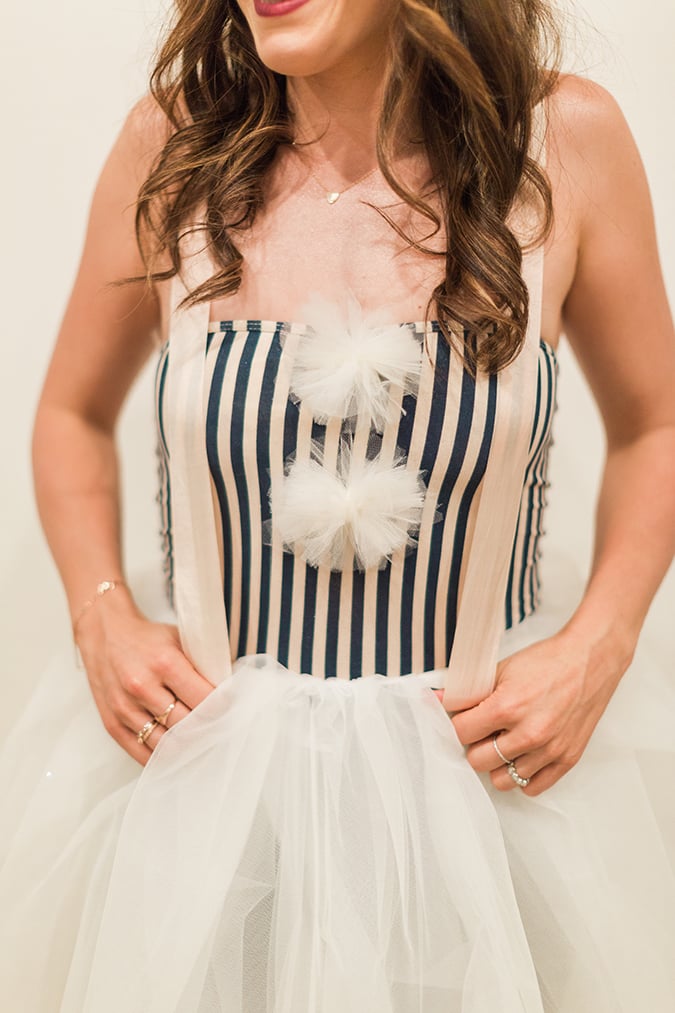This image is a close-up photograph of a Caucasian woman from her chin down to below her waist, capturing part of her highlighted brown hair and the bottom of her lips adorned with pink lipstick. She is smiling, though most of her mouth is out of the frame. The woman is dressed in a white and peach gown adorned with black vertical stripes running down the middle. The top of the dress features puffy, fluffy embellishments aligning with the black stripes, giving it a bustier-like appearance. Over her shoulders, light pink straps, resembling suspenders, add a touch of elegance. The bottom part of the dress is a thin, wispy material, akin to tulle or a tutu. She accessorizes with a heart-shaped necklace, a silver bracelet on one hand, and several rings, gold and silver, on the middle and ring fingers of both hands. Her hands rest on her waistline, and the background of the image is a simple white, keeping the focus entirely on her detailed and stylish ensemble.